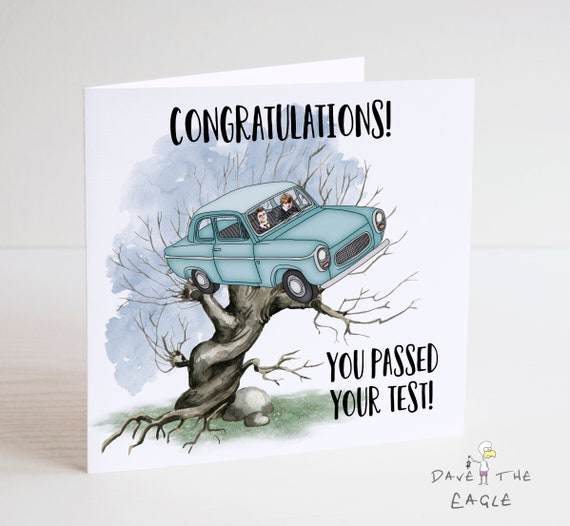This image depicts a humorous greeting card resting on a white wooden table, resembling a stock photo setup. The card features a whimsical watercolor illustration of a barren, leafless tree with an old teal blue car lodged in its branches. Inside the car, drawn in a 1950s style, sit Harry Potter and Ron Weasley, dressed smartly, with Ron appearing to be driving. The card prominently displays the message "CONGRATULATIONS! YOU PASSED YOUR TEST." in bold, black capital letters above the scene, with "you passed your test" repeated below the car. At the bottom right corner, the signature "Dave the Eagle" accompanies a cartoon caricature of an eagle holding something, adding another layer of humor to this playful congratulatory card. In the foreground, the tree stands amidst green grass and some rocks, enhancing the quirky scenario of celebrating a new driver’s success in a lighthearted, tongue-in-cheek manner.